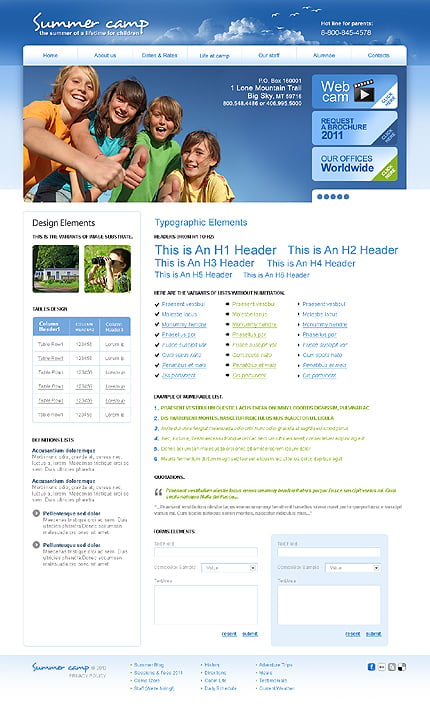The image showcases a vibrant and detailed launch page for a summer camp. The top banner is a vivid blue, transitioning to a lighter blue just below. The main portion of the page, comprising around two-thirds of the image, is a clean white, with the bottom 10% returning to the blue theme. Highlighted in elegant cursive font, the words "Summer Camp" appear in white, heralding "The Summer of a Lifetime for Children," embellished with playful clouds to the right of the phrase. 

Adjacent to this cheerful text, the page provides a hotline for parents: 800-845-4578. Just below this section, a navigation menu features neatly arranged boxes with options labeled: Home, About Us, Dates and Rates, Life at Camp, Our Staff, Alumni, and Contact.

In the midsection of the webpage, there's an engaging photograph of three children, smiling and giving thumbs up — arranged boy, girl, boy. Further to the right, the contact information is listed, providing an address: P.O. Box 16001, One Lone Mountain Trail, Big Sky, Montana, followed by additional contact details including two phone numbers.

To the right of the contact information, several actionable buttons are displayed: Webcam, Request a Brochure 2011, and Our Offices Worldwide. Below these buttons, a section labeled "Typographic Elements" appears, aimed at showcasing the webpage's construction. It includes various design instances like headers, bullet points, examples, comments, and a comment section.

Adjacent to this section, "Design Elements" is featured, illustrating different design options and potential pricing points. The webpage culminates in a sitemap section at the bottom, with links clearly marked in blue lettering.

This descriptive launch page is designed to be both engaging and informative, ensuring parents can easily navigate through crucial camp information, contact details, and additional resources.